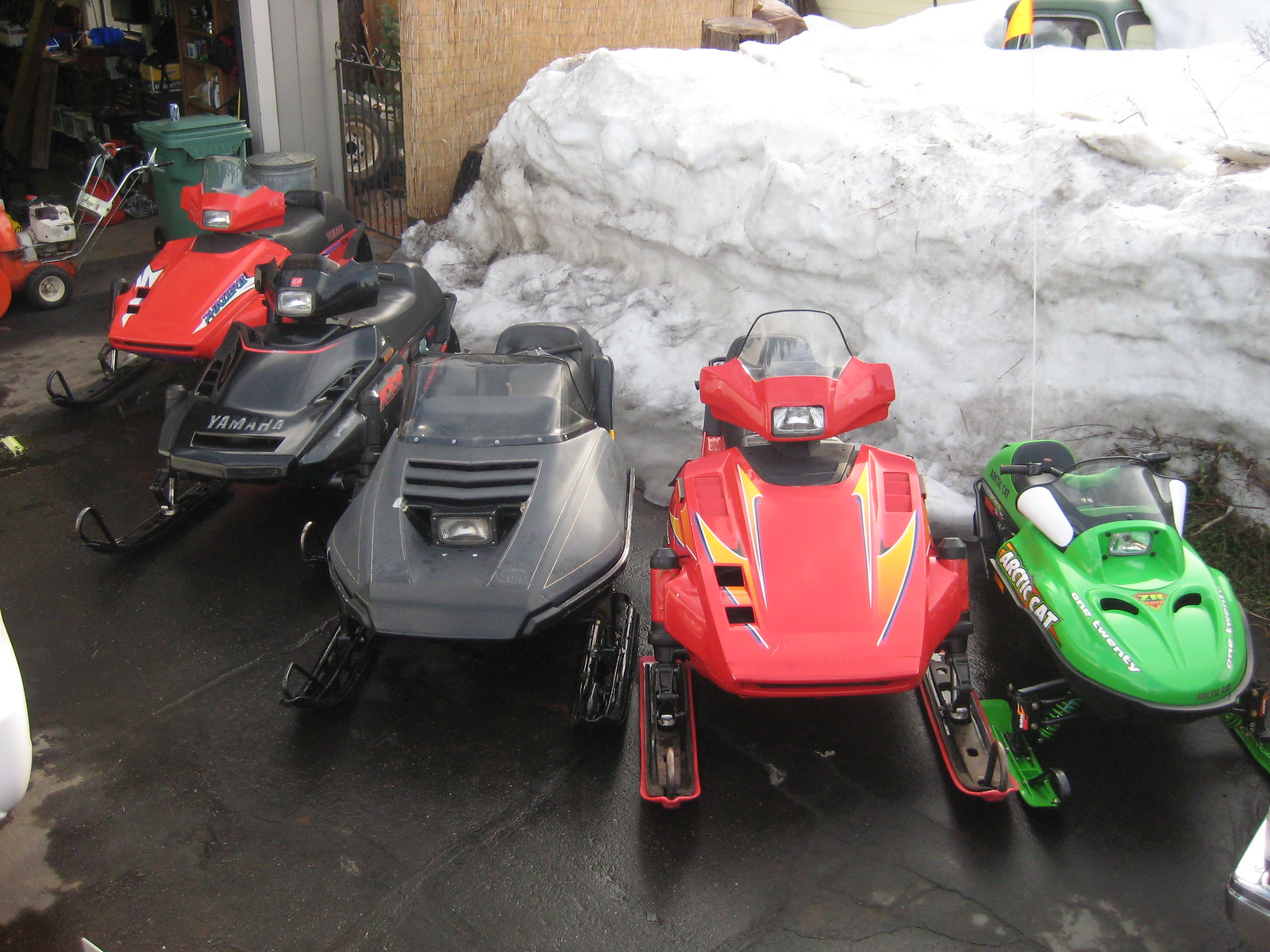The photograph captures an outdoor scene in a parking lot or garage area during the daytime. The ground is asphalt, with some areas appearing wet. Dominating the background, a large mound of snow, approximately four to five feet high, extends across the scene. In front of this snow mound, five snowmobiles are parked in a curved formation. From left to right, there's a little red snowmobile, a black Yamaha snowmobile, a medium-sized black snowmobile, a medium-sized red snowmobile, and a smaller green snowmobile resembling an Arctic Cat for a child. The upper left corner of the image reveals an open garage door, where various items such as a green garbage bin with a soda or beer can on it, a snowblower or lawnmower, and other tools or benches are visible.